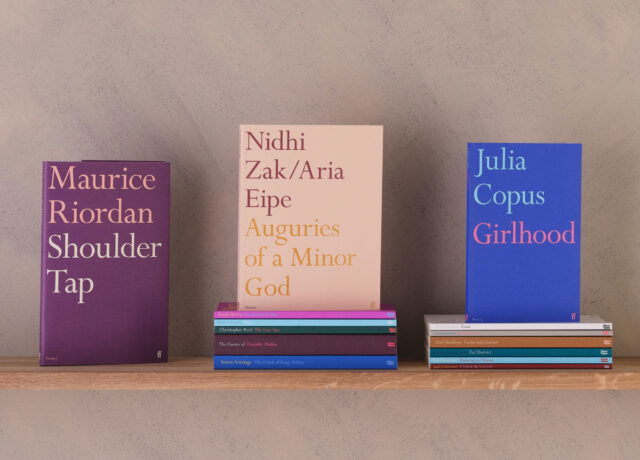This photograph showcases a light brown shelf adorned with a meticulously arranged trio of book stacks set against a gray wall. The left-most book, with a maroon cover and off-white lettering, stands proudly on its own. It is authored by Maurice Riordan and titled "Shoulder Tap." The middle stack comprises five horizontally laid books of assorted colors, including blue, maroon, green, turquoise, and pink, with a tan book positioned vertically on top. This book, with its pale background and red and yellow text, is titled "Auguries of a Minor God" by Nidri Zak. To the right, the last stack consists of six books laying flat, topped with a bright blue-covered book featuring light blue and pink lettering. Authored by Julia Copas, it is titled "Girlhood."